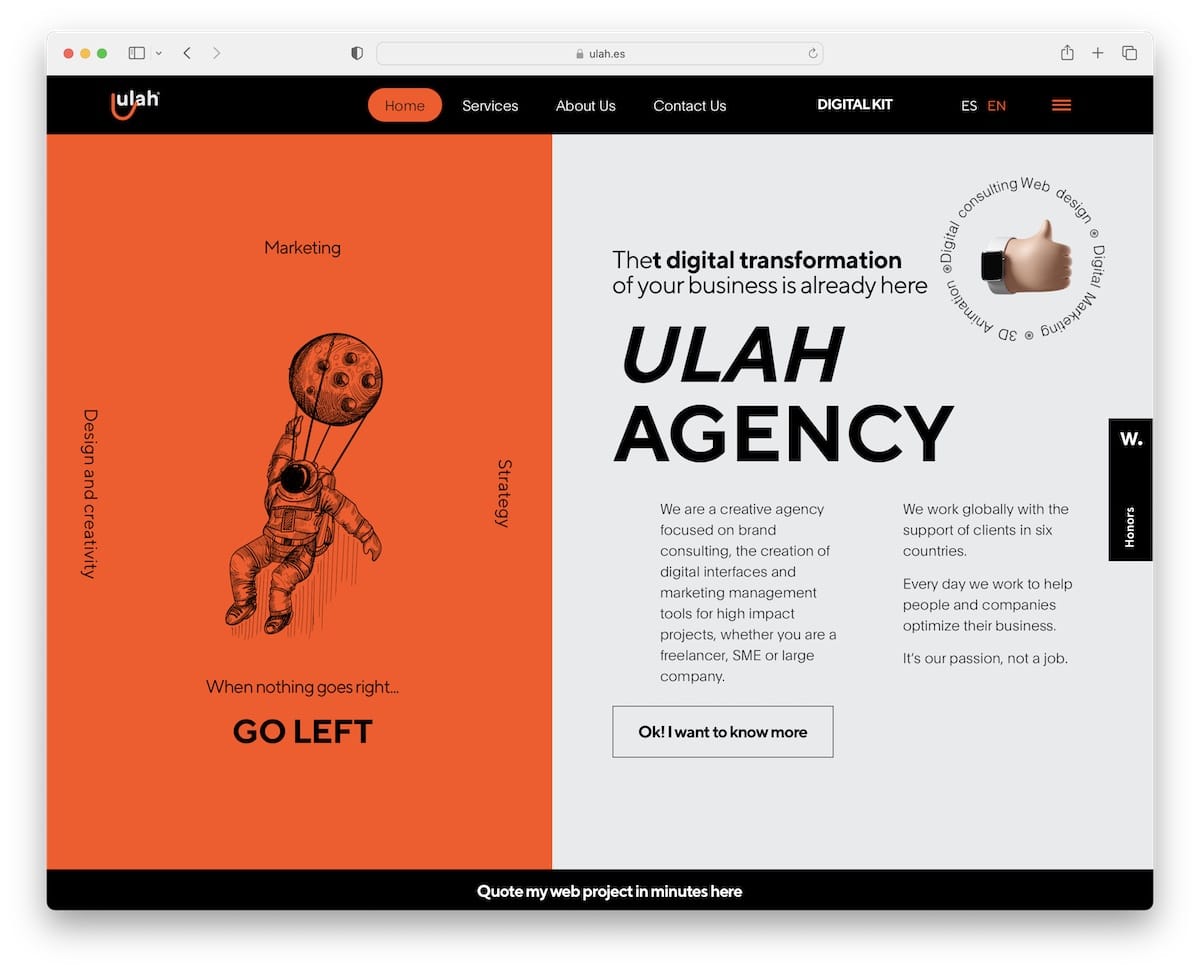This digital image depicts a sophisticated web page from a consulting agency, EULA. The page features a black header at the top that lists navigation links: Home, Services, About Us, Contact Us, Digital Kit, and ESEN. The left half of the screen is vibrant with a red-orange background, featuring an astronaut with a black helmet and a moon tethered to him by four strings, seemingly skydiving. Text on the left side reads "Marketing," "Design and Creativity," and "Strategy." Beneath the astronaut, a motivational quote says, "When nothing goes right, go left." The right half contrasts in white, with a corner emblem and an image resembling a thumbs-up. Key statements are written in black, proclaiming, "The digital transformation of your business is already here," followed by "EULA Agency." Additional text emphasizes their focus on brand consulting, digital interfaces creation, and marketing management tools for high-impact projects, catering to freelancers, SMEs, and large companies. Further down, it mentions EULA's global clientele from six countries, and their dedication to optimizing businesses with passion. A black box with an unreadable white text is present on this side. At the bottom of the page, a white button with black text reads, "OK, I want to know more," above a black stripe stating, "Quote my web project in minutes here."